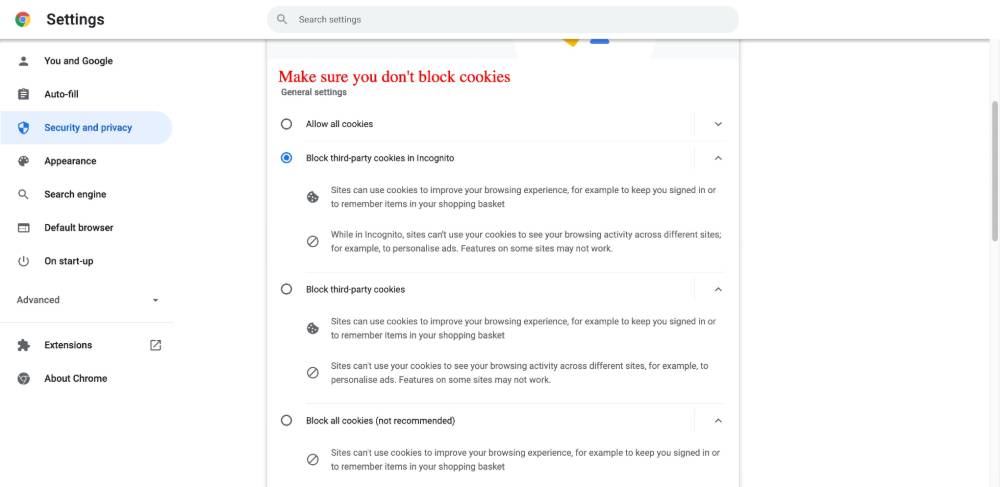The image depicts a webpage displaying the settings interface of Google Chrome. In the upper left-hand corner, there is the distinct Google Chrome icon followed by the word "Settings" in bold black font. To the right of this title, centrally aligned, lies an oval-shaped search bar in a light gray shade, containing the placeholder text "Search settings" and a magnifying glass icon on the far left of the bar.

On the left side of the interface, there is a vertical menu of icons and labels starting with "You and Google," followed by other options such as "Autofill," "Security and privacy" (which is highlighted in a light blue shade), "Appearance," "Search engine," "Default browser," and "On startup." Below these, a thin line demarcates the section before the options continue with "Advanced," and further down lists such as "Extensions" and "About Chrome," each accompanied by their corresponding icons. Near the "Extensions" label, a small box with an arrow inside is visible.

Under the search settings bar, there's an advisory note stating "Make sure you don't block cookies," followed by relevant options concerning cookie settings. The current configuration indicates that "Allow cookies" is active and "Block third-party cookies in Incognito" is checked. Additional selections present but not recommended include "Block third-party cookies" and "Block all cookies."